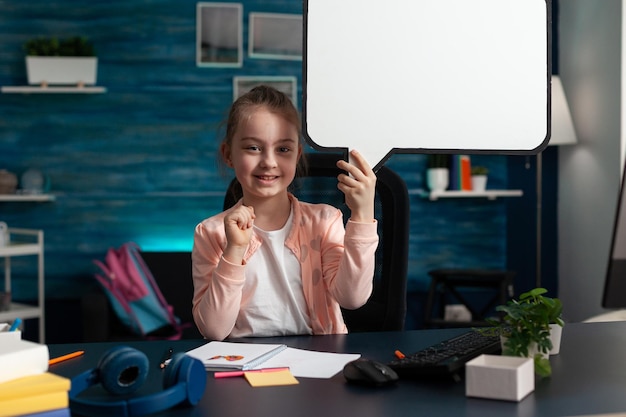In the image, a young girl, roughly nine years old, is sitting at a black desk in a room with a blue wall. She has a cheerful expression and is dressed in a pink sweater over a white t-shirt. Her brown hair is neatly pulled back into a ponytail. In her right hand, she holds up a whiteboard shaped like a comic book speech bubble, ready to be written in. 

The desk is adorned with various items, including a small green plant in a white box, a pair of blue headphones, and an open journal displaying a pink drawing. Nearby, a yellow notepad sits alongside a white notebook with a pink pen. A black mouse and keyboard are also present. The background features white shelving decorated with plants and miscellaneous items, a trio of small pictures grouped together, and a distant pink and blue backpack, hinting that she is likely at home.